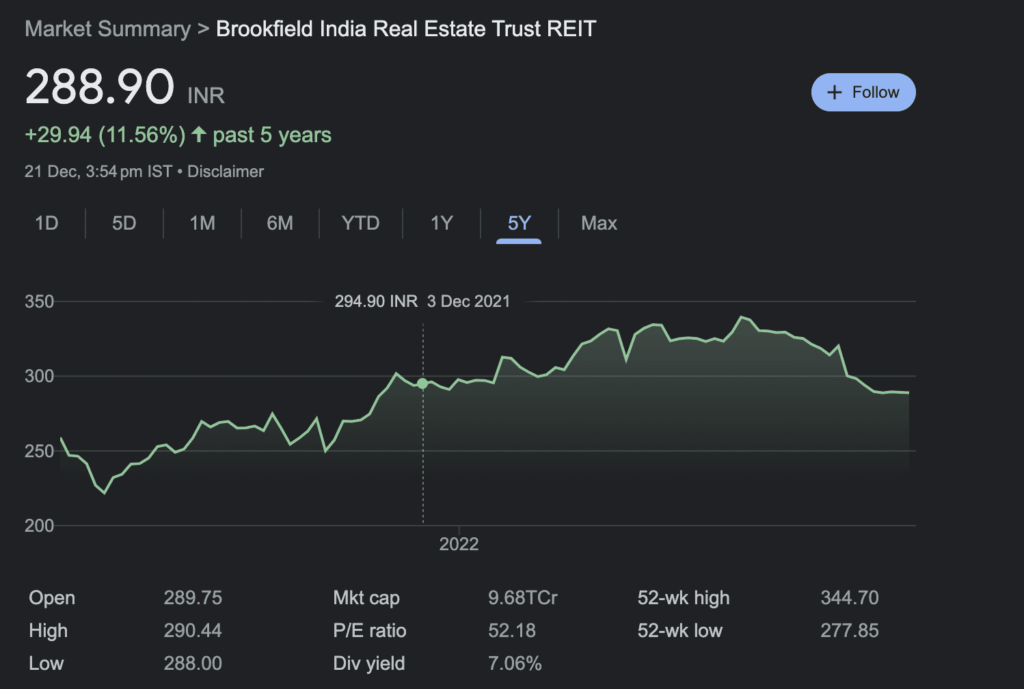The image displays a detailed market summary for Brookfield India Real Estate Trust (REIT) in the top-left corner, highlighted in gray. An arrow pointing right accompanies the title. Listed next is the value "288.90" in bold, followed by "INR" in uppercase on the same row. Below this, a green plus sign indicates "29.94," representing a change of "11.56%" within parentheses. A green arrow next to these figures points upward, denoting positive growth over the past five years.

The central area features a detailed graph. The y-axis is labeled with increments descending from 350 to 200. The green trend line on the graph initiates near the 250 mark. A notable dip occurs, bringing the line close to the 200 mark, after which it stabilizes with minor fluctuations, indicated by subtle up-and-down movements. At the 300 mark, the graph is highlighted by a green circle, signifying a key data point. The line then continues an overall upward trajectory, with minor downwards fluctuations toward the right of the graph. Accompanying the graph, the date "3 December 2021" is indicated, with the value "294.90 INR" displayed at the top.